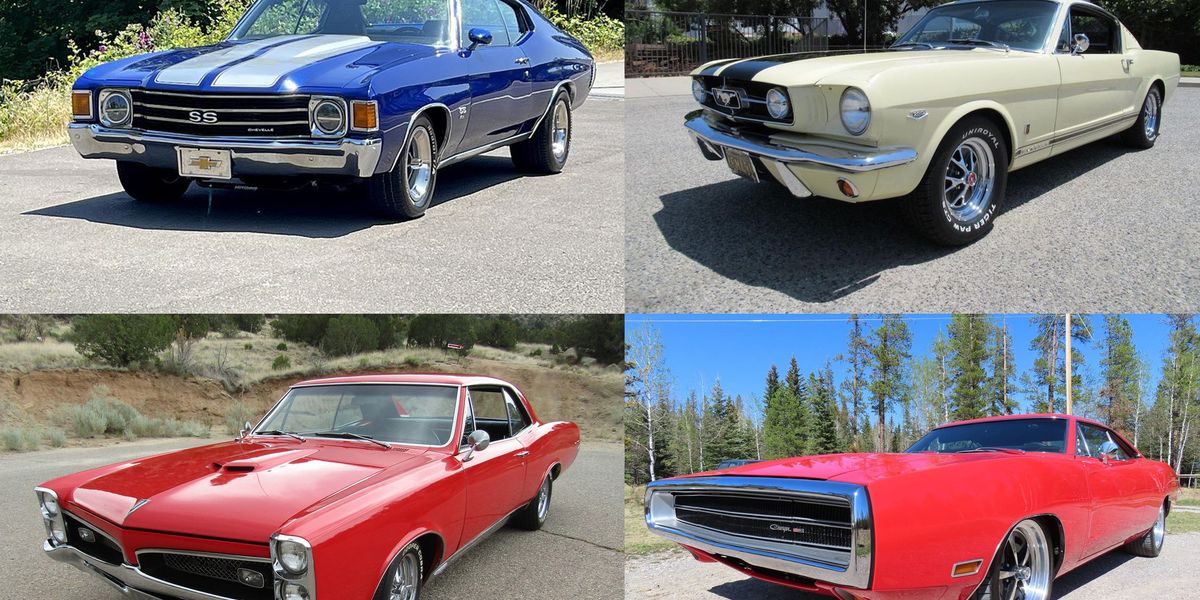The image is a grid of four distinct photos showcasing meticulously restored American muscle cars from the 60s and 70s. The top left photo features a navy blue Chevrolet SS Chevelle with silver racing stripes on its hood, distinguished by its chrome accents and SS badge on the front grille. The top right photo captures the front left headlight of a cream-colored mid to late 60s Ford Mustang Fastback, detailed with black racing stripes and a horse badge on its squarish bonnet. The bottom left image showcases a dark cherry red Pontiac GTO with a prominent hood scoop and vertical headlights. The bottom right photo presents a light red Dodge Charger, characterized by its wide hood and elongated rectangular front grille. All cars are set against a backdrop of light gray pavement, with green foliage and dark evergreen trees enhancing the scene. Sunlight illuminates the tops of the cars, except for the vehicle in the bottom left corner, creating a dynamic contrast in brightness across the photos.